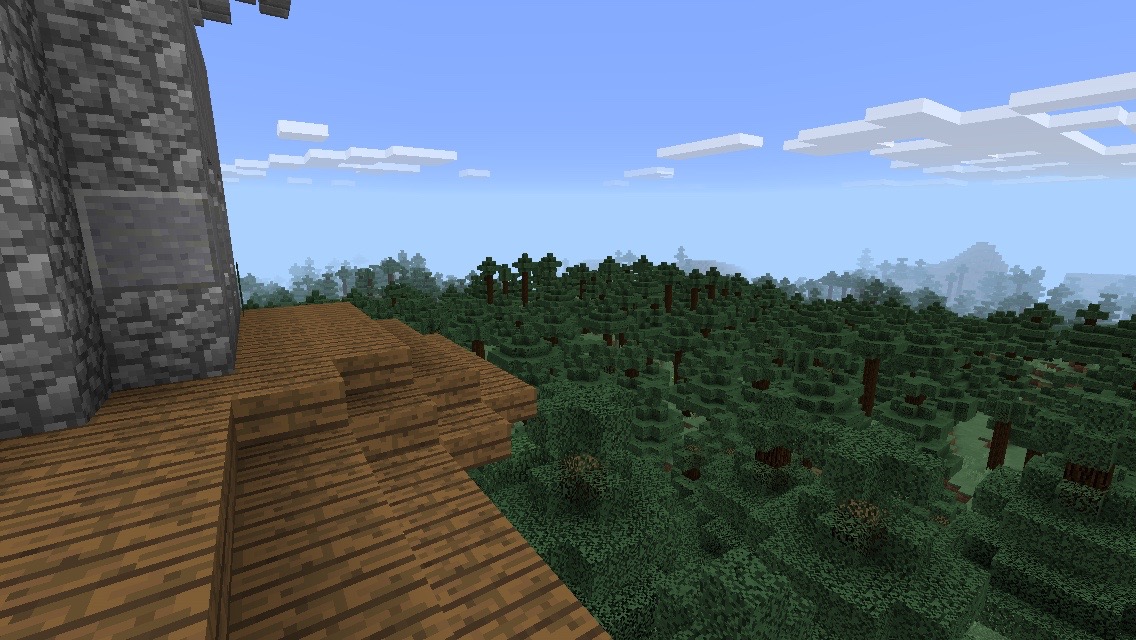This captivating image appears to be a scene from a video game, characterized by its unique and stylized graphics. The sky is a vivid blue, dotted with clouds that are intriguingly constructed from square shapes, reminiscent of Lego blocks pieced together in an artistic mosaic. Dominating the foreground is a grand stone building, exuding an air of ancient strength and stability. The structure features distinct wooden steps with planks oriented perpendicularly rather than lengthwise, providing a charming and rustic feel. The steps lead up through three visible levels, each accessible by a short flight of about four steps. Surrounding the stone edifice, a lush multitude of green trees fills the scene, their vibrant foliage contrasting beautifully with the sturdy stonework. In the distance, towering mountains stretch up towards the sky, adding depth and a sense of majesty to the landscape. The juxtaposition of the odd, geometric clouds above with the natural, verdant surroundings below creates a strikingly whimsical atmosphere.